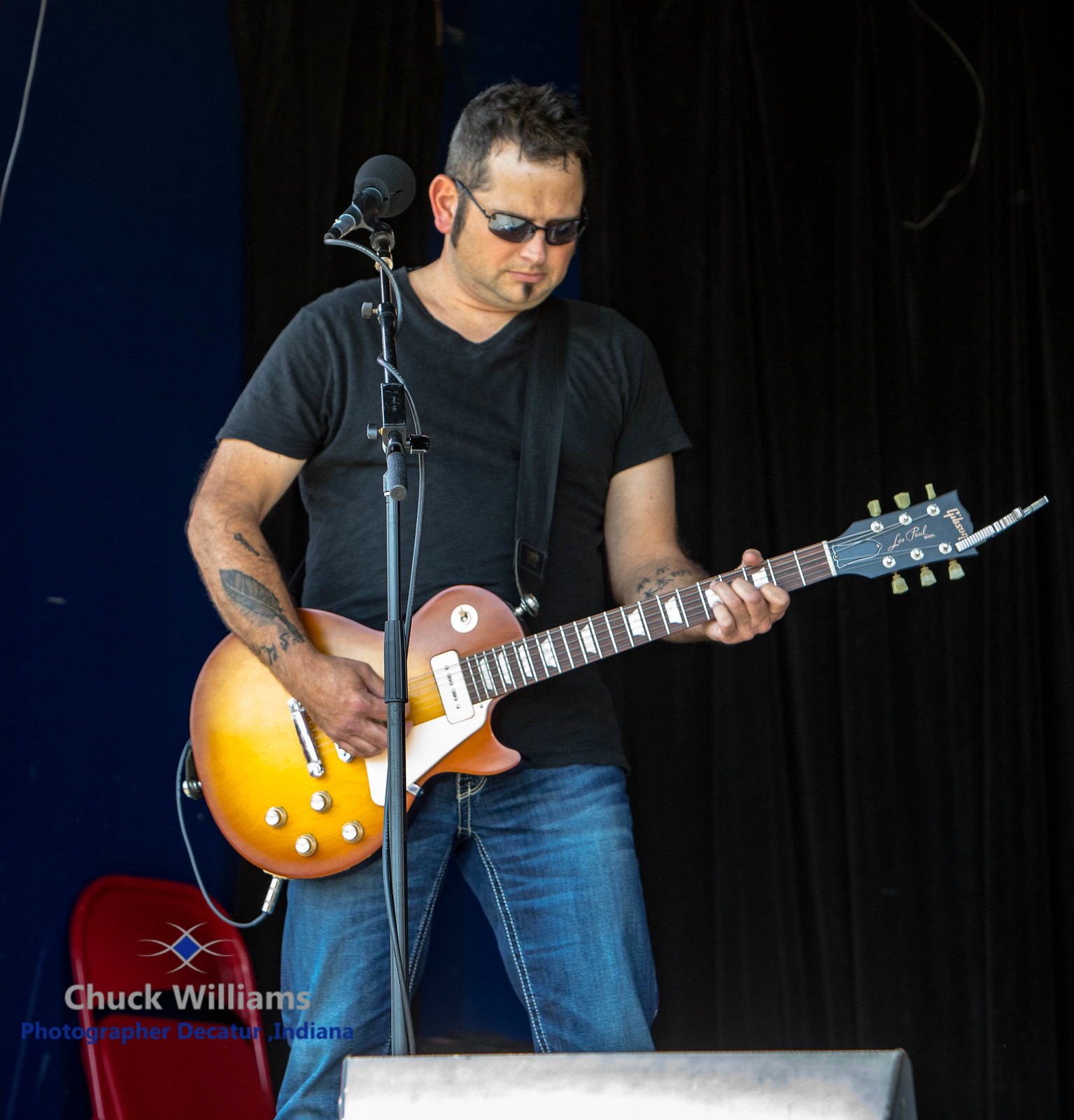A man stands on a stage, intently playing a Gibson Les Paul guitar with a sunburst finish, characterized by its orange and yellow hues and detailed with tuner pickups. He wears black sunglasses, a black short-sleeved V-neck T-shirt, and blue jeans, which showcase his forearm tattoos. His short black hair is accompanied by a small goatee and pronounced long sideburns. The scene is set against a black curtain with a blue wall to the left. A red folding chair leans against the curtain behind him, and a black, box-shaped speaker faces him at the bottom of the image. In front of him, a black microphone on a stand captures the moment, with a black guitar strap securing his instrument. A subtle caption in the lower left corner reads "Chuck Williams."